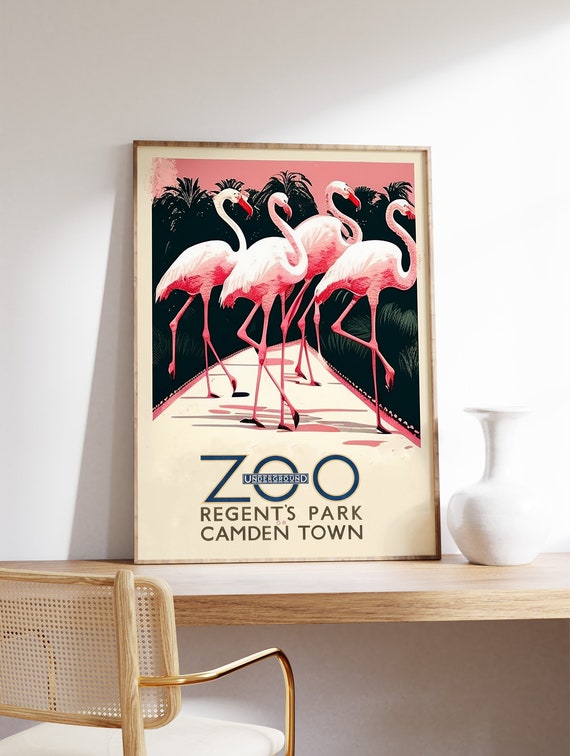The image showcases a framed poster in a brown wooden frame, prominently displaying four pink flamingos with their legs lifted, against a background of blackened palm trees and a pink sky. The poster, leaning against a white wall on a thick, light wood table, reads "Zoo Regents Park Camden Town" in black text, with a small, unreadable detail within one of the O's. To the right of the poster sits a minimalist white vase, adding to the overall barren aesthetic. In the foreground, there's a chair with a cane mesh back, brass metallic armrests, and a white seat cushion, positioned next to the table. The scene evokes a modern, clean setting that draws attention to the vibrant, stylized depiction of the flamingos marching along a path in the poster.